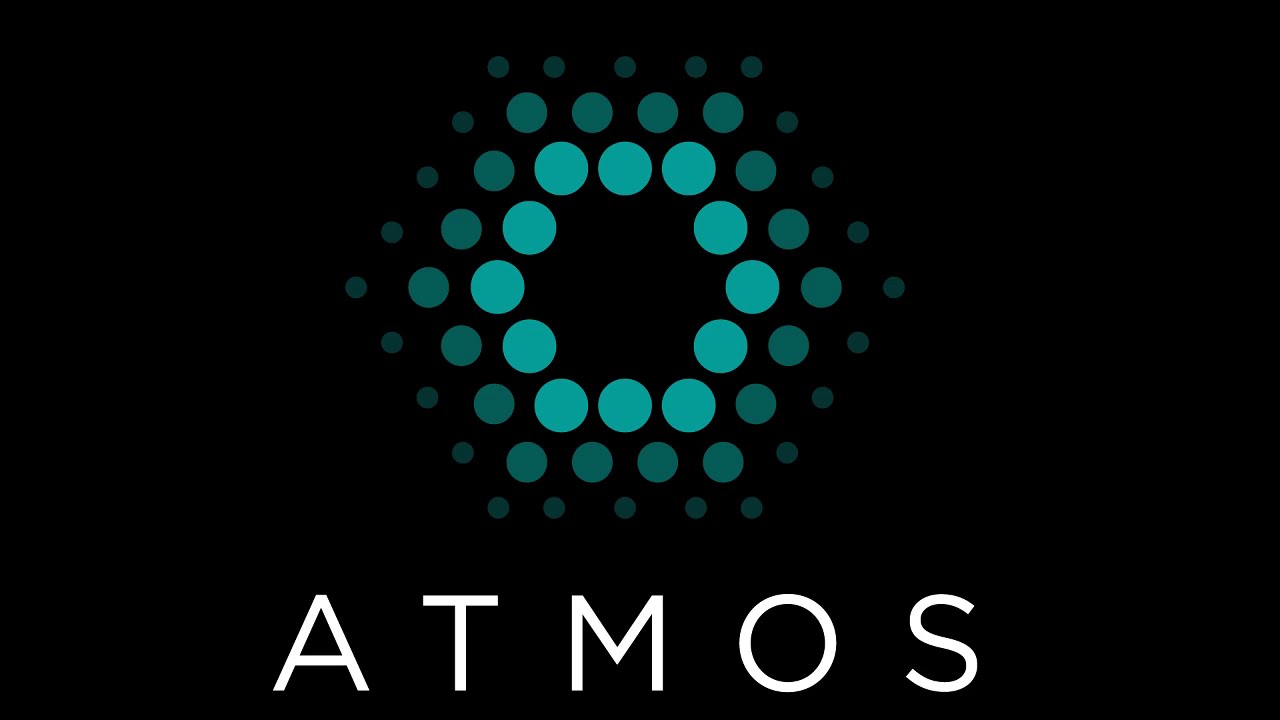This image features a sleek, black background resembling that of an advertisement or business card, underlining a sense of modernity and minimalism. At the bottom of the image, the word "ATMOS" is prominently displayed in bold, capitalized, white letters, centered perfectly. Above this text is an intricate company logo, consisting of a series of concentric geometrical shapes, likely hexagons. The design begins with a central hexagon made up of interconnected, bright turquoise dots. Surrounding this are two additional hexagonal patterns, each progressively darker in shade and fading as they extend outward. The outermost hexagon is composed of smaller, dark turquoise dots, creating a sense of depth and complexity. The cumulative effect is one of a dynamic, interconnected network, symbolizing perhaps the essence of the company's identity.